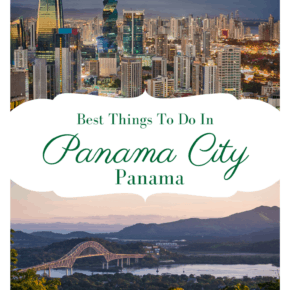This image appears to be an element from a web page, with a nearly square shape that is slightly taller than it is wide. The design features two photographs, one at the top and another at the bottom, with a white background in the center that resembles the form of a cloud. The central section includes light greenish-gray font that reads "Best Things to Do in Panama City, Panama," with "Panama City" prominently written in a large, script-like font resembling handwriting.

The top photograph showcases a vibrant cityscape viewed from a high vantage point, capturing numerous tall skyscrapers. The image is taken during a transitional time of day, either daybreak or twilight, as evidenced by the illuminated windows of some buildings casting a warm glow.

The bottom photograph depicts a serene landscape with a distant mountain range characterized by purplish hues. The sky is painted in shades of pink, suggesting it is either at sunrise or sunset. In the foreground, a river flows gently, spanned by an elegant bridge. The combination of these elements crafts a compelling visual representation of Panama City's urban and natural beauty.